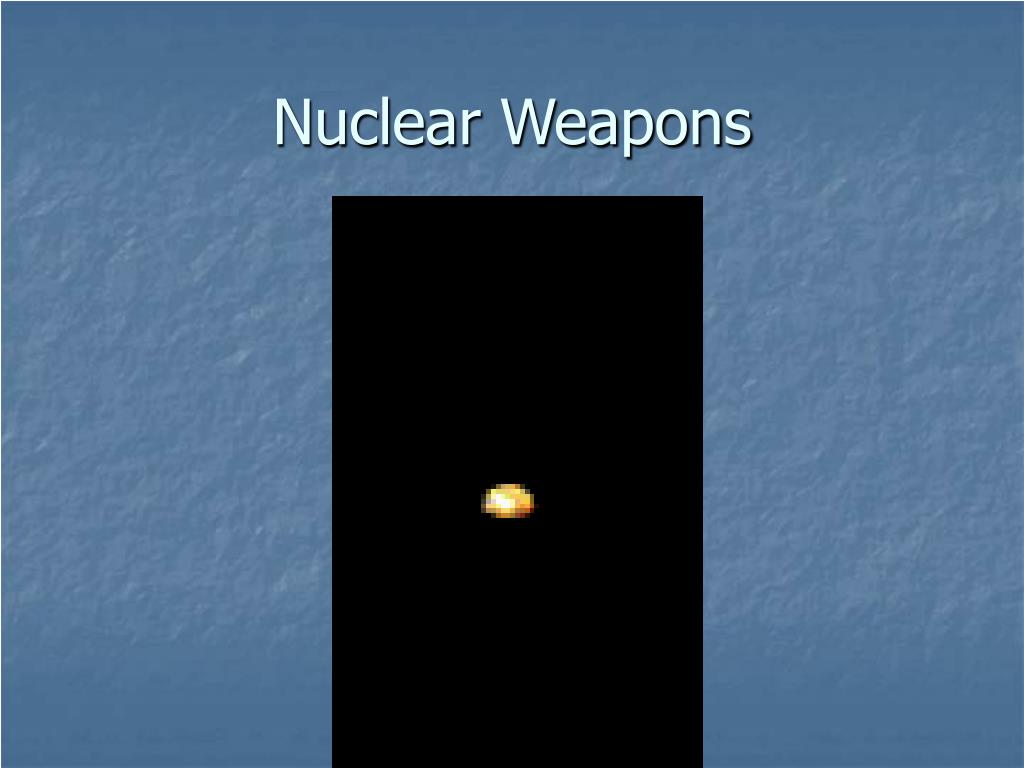The poster features a blue background with a rough, uneven texture that gradually smooths out towards the bottom. In the center of the poster, there is a black rectangle. Above this black rectangle, the text "Nuclear Weapons" is prominently displayed in light powder blue letters, with the initials "N" and "W" capitalized. Within the black rectangle, a shining golden-yellow oval object with a pixelated, digitized appearance is centered, standing out vividly against the black backdrop. The exact nature of this golden object is unclear, resembling either a nuclear weapon, a prize, or an item from a video game.